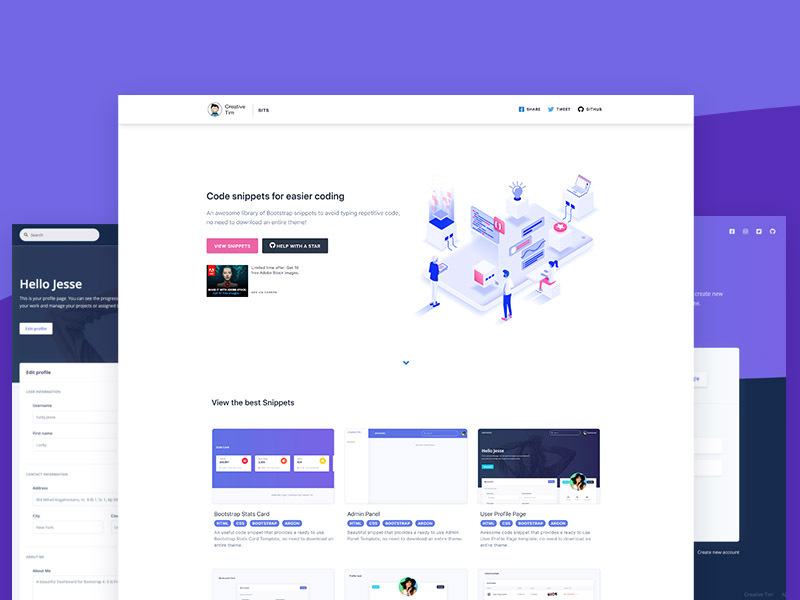The image captures a screenshot from a desktop or laptop displaying two overlapping windows. The background of the desktop features a wallpaper with medium and light purple waves. 

The rear window, partially obscured by the front window, has a visible left-hand section that greets "Hello Jesse" with additional illegible text below. Underneath, there is a button followed by the text "Edit Profile" which appears to offer five dropdown menu options.

The foreground window prominently displays the heading "Code snippets for easier coding." Beneath this heading, there are two lines of text that are unreadable, followed by a pink button labeled "View Snippets." Adjacent to this button, on a black tab with white text, the word "Help" is visible, potentially accompanied by an asterisk.

Below the "View Snippets" button is an image of a woman's face, with text to its right. Further to the right, there is a graphical representation of people working in an office, suggesting a collaborative or professional environment.